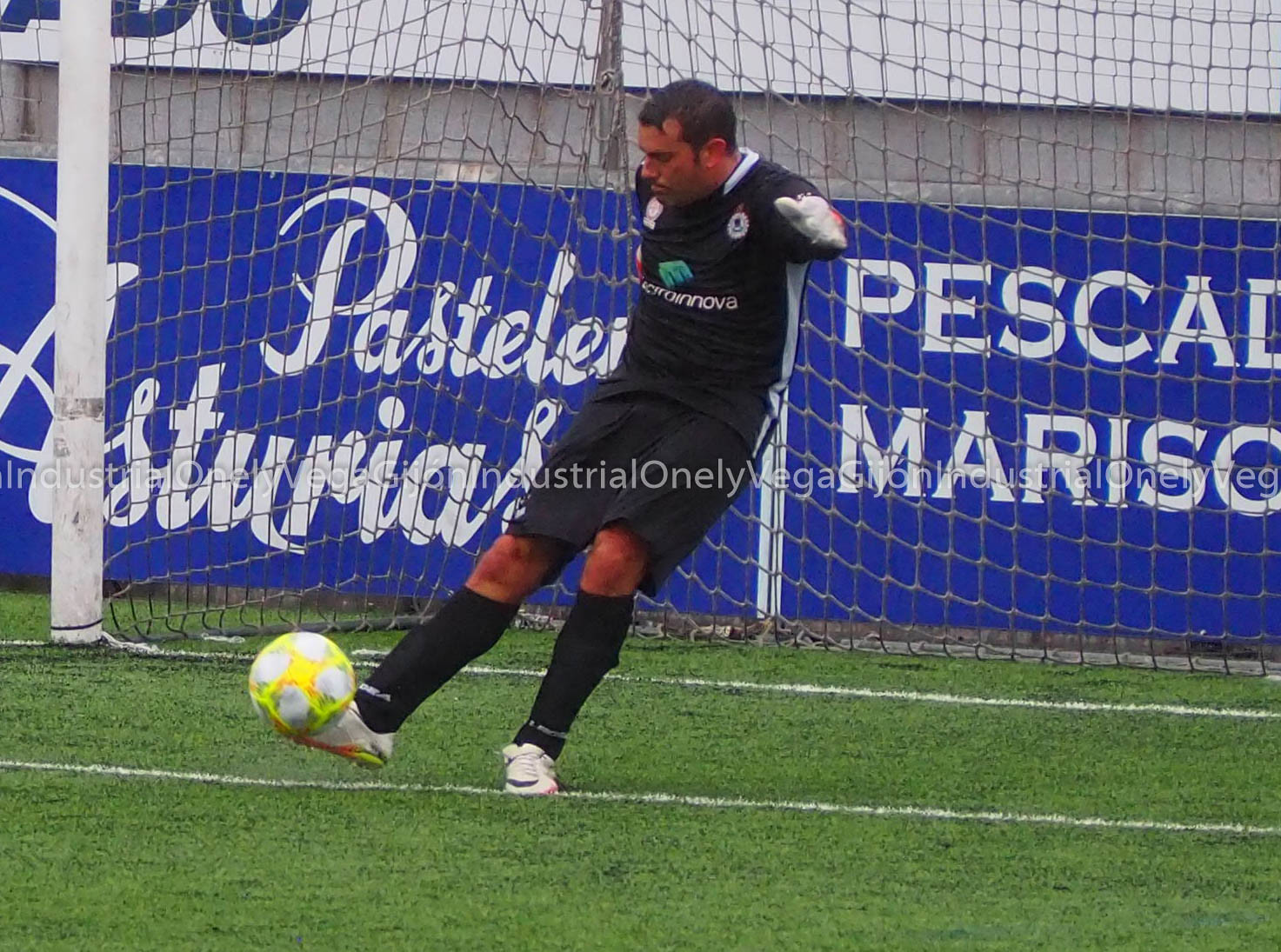A dynamic and detailed image captures a soccer player in mid-action, his right foot poised to kick a soccer ball. The solitary figure stands out on a vivid green soccer field, with prominent white stripe markers underfoot. He is clad in a black jersey adorned with an insignia featuring white lettering and a green symbol, complemented by white gloves, black shorts, black socks, and white shoes. His arms are extended, suggesting a follow-through motion, and his focus is intently on the ball. Behind him, a substantial goal net spans the width of the image, partially obscuring a large blue sign that runs the length of the background. The text on the sign is partially hidden but includes terms like "Pastel," "Asturias," and "Mariso." His position, right in front of the net, along with his distinctive outfit, suggests he might be the goalie. His dark hair contrasts against the backdrop, further highlighting his intense concentration on the play.